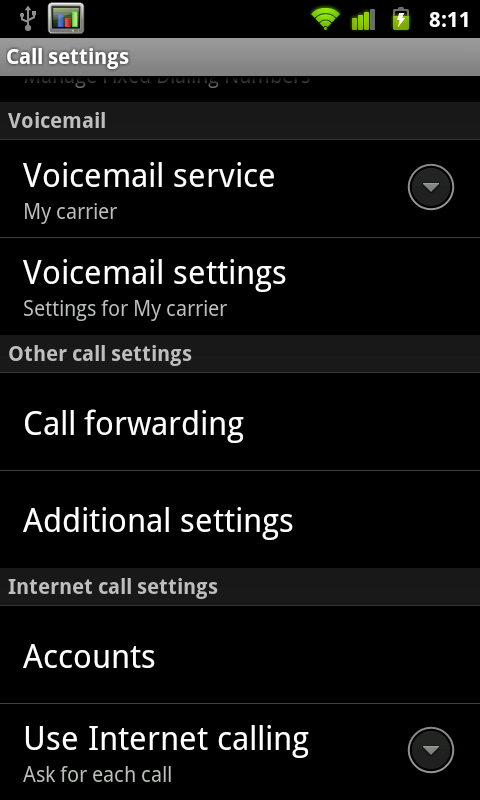The image is a screenshot of a mobile device displaying the "Call Settings" menu. 

At the very top, the standard mobile status indicators are visible, featuring green Wi-Fi and battery icons. On the right side, the time is shown in white, reading 8:11. On the left side, two icons are present: one resembling the top of a trident, and the other depicted as a small monitor displaying a bar chart with a medium-sized blue bar, a shorter red bar, and a taller green bar.

Below this status bar, there is a thin, gray rectangular header with the words "Call Settings" displayed in white on the left. The main section of the screen has a black background with several headings and options in white and gray.

The first section is labeled "Voicemail" in gray. Underneath, the option "Voicemail Service" is listed with "My Carrier" displayed beside it. To the right, there is a gray circle with a light gray upside-down triangle. A thin separator line divides the next option, "Voicemail Settings," which includes a smaller gray font description, "Settings for My Carrier."

Following this, another gray rectangular heading says "Other Call Settings." Two options are listed below: "Call Forwarding" and "Additional Settings," both in white.

The final section is labeled "Internet Call Settings" within a gray box. Two options are listed underneath: "Accounts" and "Use Internet Calling," the latter having a smaller gray subtext, "Ask for Each Call." On the right side of this option is a dark gray circle with an upside-down light gray triangle.

Each section is clearly delineated with gray headings and borders, providing an organized and straightforward layout for managing call settings on the mobile device.